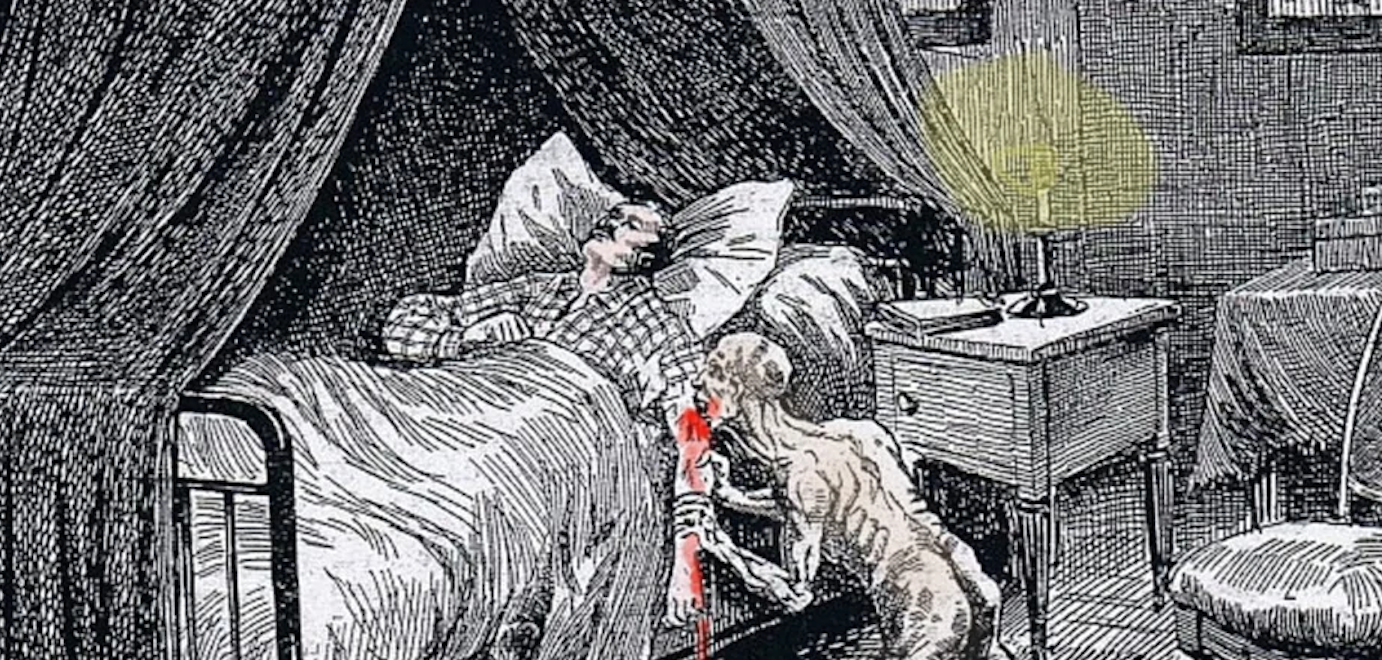This black and white illustration depicts a haunting scene of a man sleeping in a metal-framed twin bed, propped up on a large pillow, and covered with a plaid blanket that's draped over his belly and part of his legs. He wears plaid pajamas and is partially covered by a netting. To the side of the bed, a bald, nude, skeletal figure kneels on the floor, biting the man's arm. Red blood can be seen dripping from the man's arm and smeared on the skeleton's face. Nearby, a nightstand holds an illuminated candle emitting a yellow glow, while a book rests beside it. Adjacent to the nightstand, there is a chair and a small table also holding some books. The eerie nature of the scene, combined with the mixed textures and muted shading of the drawing, suggests that this may be depicting some kind of nightmare or unsettling dream.